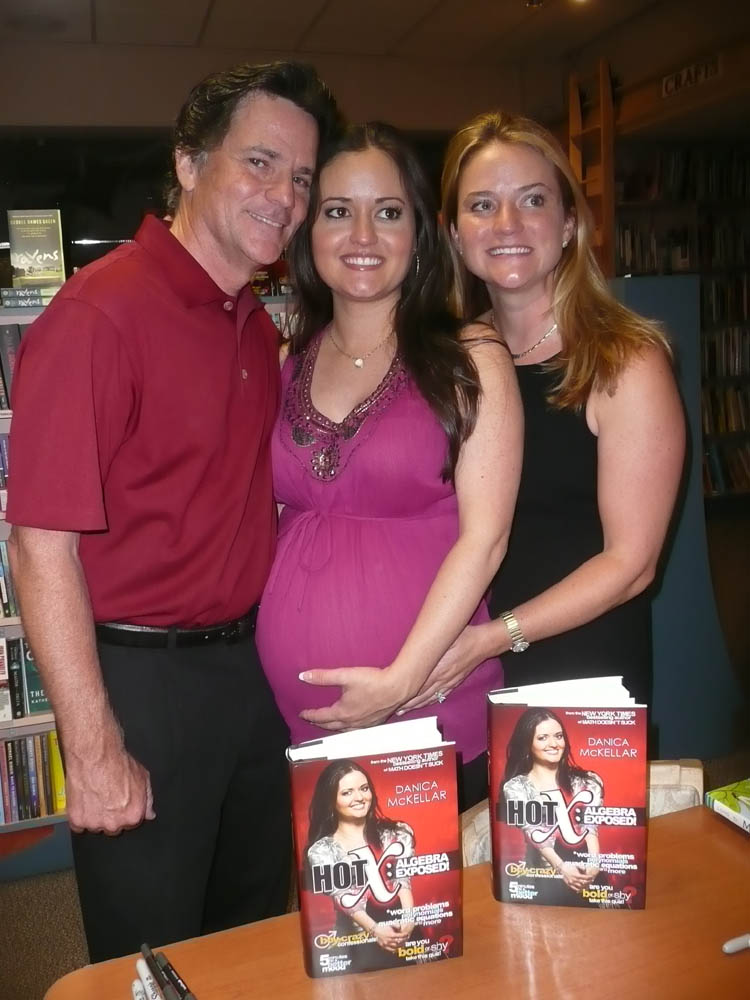The image, taken indoors, features three people standing amidst bookshelves. At the center of the photo is a pregnant woman with long straight brown hair, wearing a pink V-neck top and a necklace. This woman appears to be Danica, who was an actress on the TV show "The Wonder Years." She has her hand on her stomach and is smiling warmly. To her left stands another woman with long blonde hair in a black sleeveless dress, also with her hand on Danica's stomach, adorned with a watch on her wrist. On Danica's right side is a man with wavy brown hair, wearing dark gray pants and a red short-sleeved dress shirt. He is also smiling and has his arm around Danica. In front of them is a table displaying two copies of a book titled "Hot X: Algebra Exposed," with a cover featuring Danica. The scene is likely inside a bookstore, suggested by the surrounding shelves filled with books.